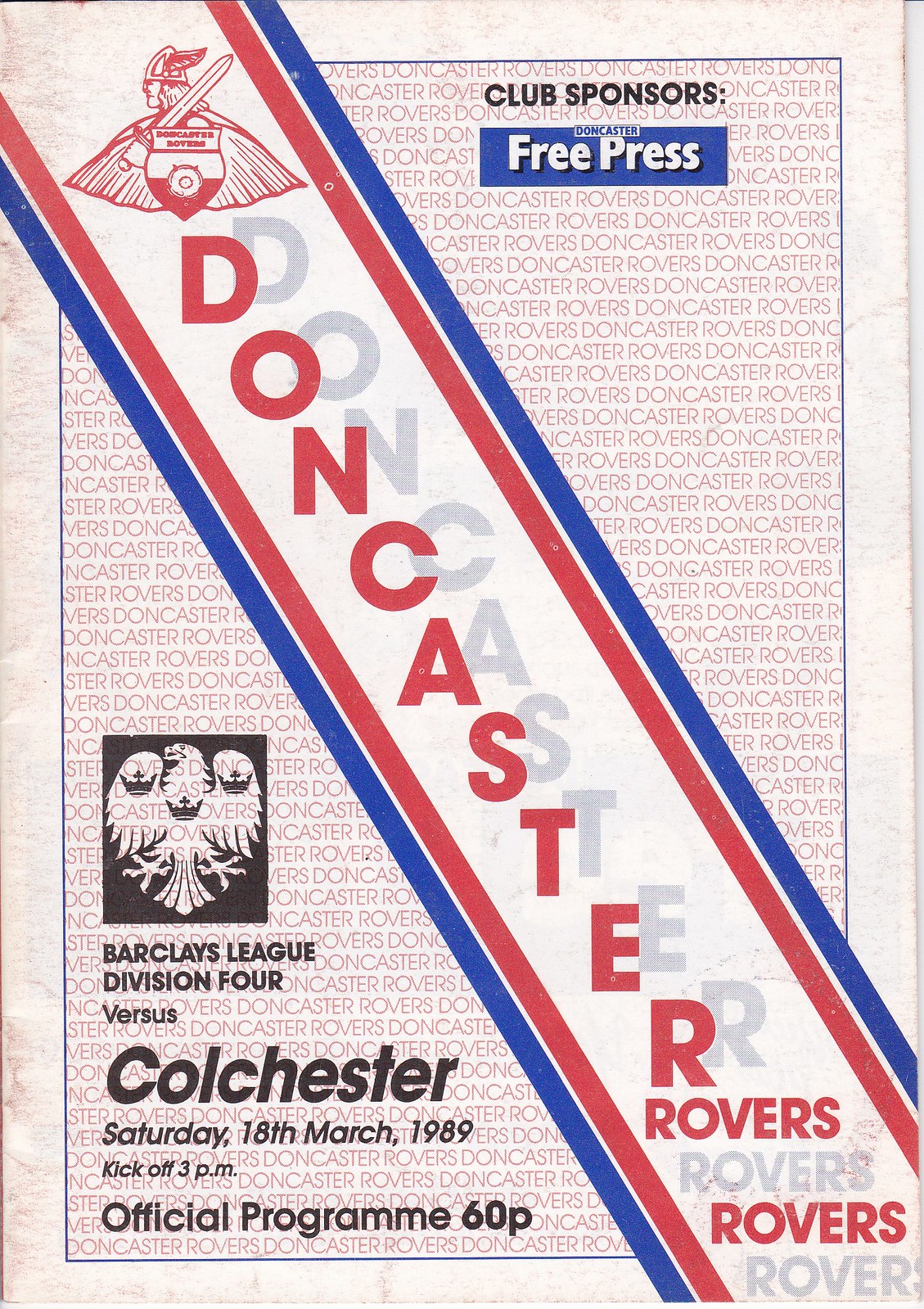This is a faded vintage cover of an old British football program for the Doncaster Rovers. A red and blue diagonal stripe runs from the top left to the bottom right, emblazoned with the name "Doncaster Rovers" in red. The background behind this stripe repeatedly features "Doncaster Rovers" in faded red writing. In the top left corner of the stripe, there's a red-outlined Viking logo, depicting a helmeted figure with wings, holding a sword and sporting a cape. Below this, the text reads "Club Sponsors" in bold black, with "Doncaster Free Press" in white set against a blue background. The bottom left quadrant outside the stripe details the match information: "Barclays League Division Four, versus Colchester, Saturday, 18th March, 1989, kickoff, 3pm, official program, 60p," alongside an emblem resembling a bird with crowns, outlined in black. The edges of the cover display a vintage white, aged to brown.